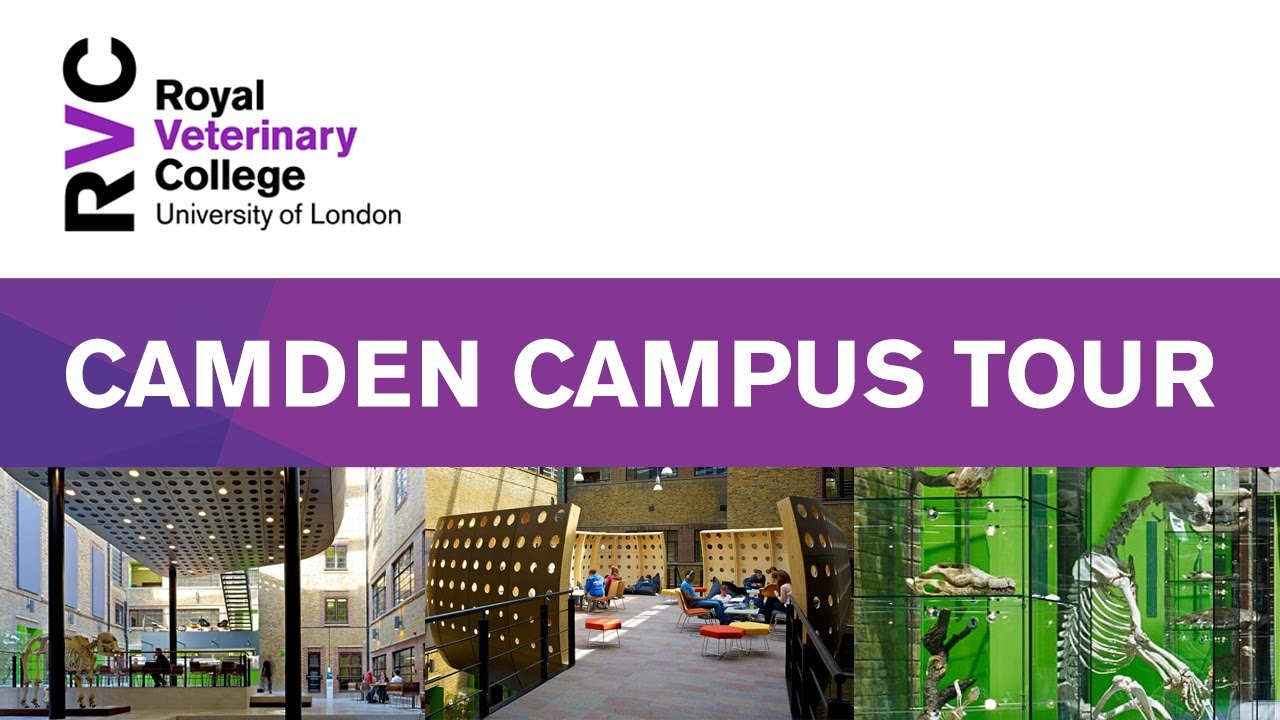The image appears to be an advertisement, possibly from a website, for the Camden Campus Tour of the Royal Veterinary College, University of London. At the top left, the logo "RVC" of the Royal Veterinary College is prominently featured, with the letters 'R', 'V', and 'C' in black and purple. Adjacent to the logo, the institution's name, "Royal Veterinary College, University of London," is displayed in standard text.

Dominating the center of the image is a large banner with a purple background and bold white lettering that reads "Camden Campus Tour." Below this main title, there are three distinct photographs that provide visual snippets of the campus. The left photograph showcases an outdoor structure with a tall overhead area featuring a roof with multiple holes. The middle image appears to show some wall-like structures with circular designs, while the rightmost photograph depicts a display of fossils and bones, possibly indicating a museum exhibit. The overall brochure cover is vibrant with a mix of purple, green, and brown hues, reflecting various aspects of the campus environment.